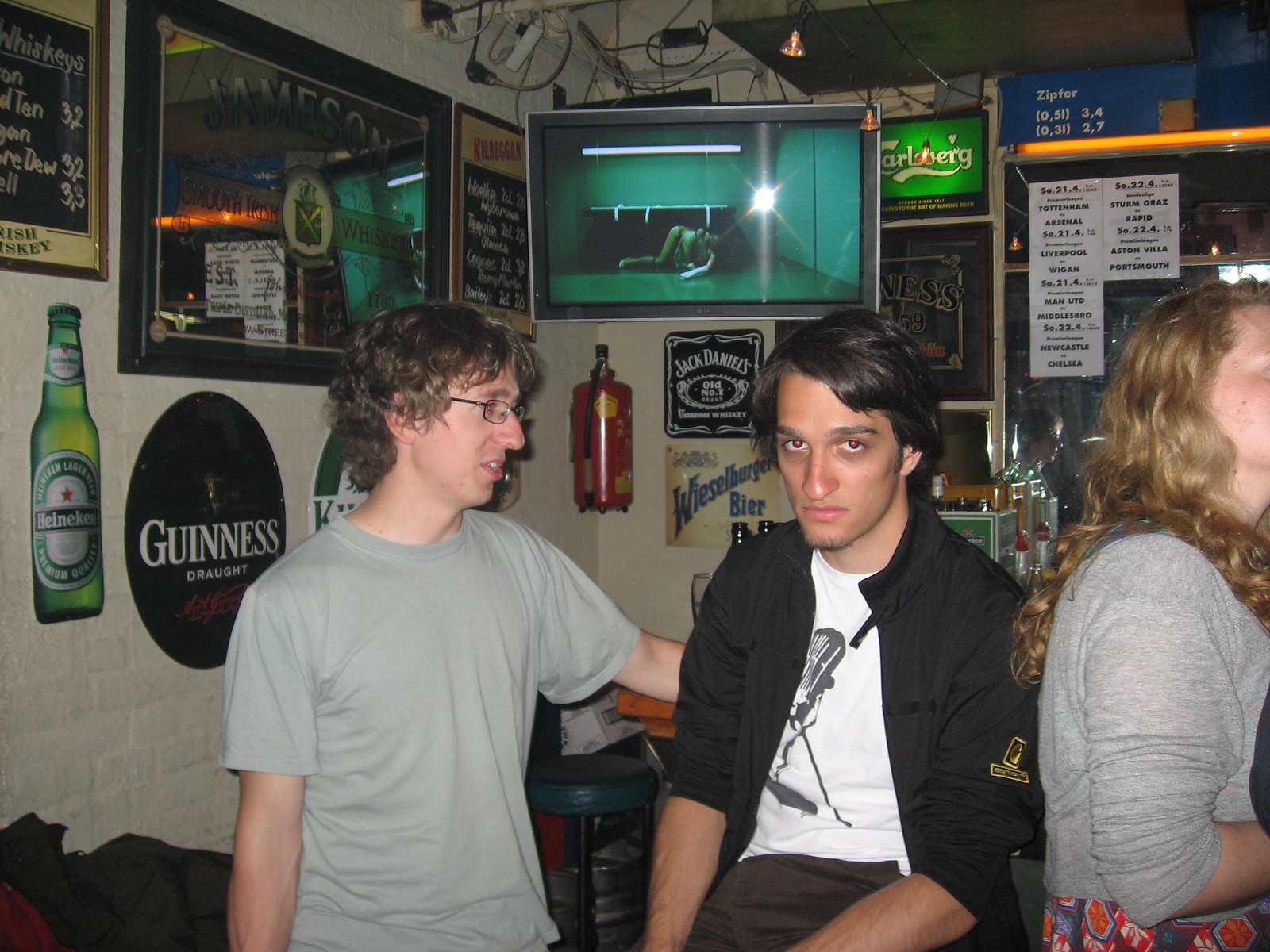In this detailed image of an Irish pub, the scene is filled with lively and eclectic décor against white brick walls that are cluttered with a variety of signs advertising drinks and sports teams. Prominently featured are signs for Heineken, Guinness, Jack Daniels, and Jameson Irish Whiskey, with a large etching for Jameson Scott Smooth Irish Whiskey on the left wall. A crowded bar area is the focal point, showcasing two young men among a trio seated at the bar, seemingly college students enjoying their evening. 

The young man on the left has curly hair, glasses, a strong nose, and wears a gray t-shirt, engaged in conversation. The central figure, with shaggy dark hair, a slightly darker complexion, and a goatee, sports a white t-shirt featuring an illustration of a microphone, layered under a black button-up shirt. He offers a serious pose directly at the camera. Just visible is a woman in a gray shirt sitting next to them. Behind them, a TV screen in the top corner, surrounded by a tangle of wires, displays a horror movie scene of a woman on the floor of an insane asylum. Adding to the ambiance, a Genesis draft beer sign, a Wells Burger beer sign, and various other signages contribute to the colorful chaos that characterizes this quintessential pub interior. A large fire extinguisher is noticeable in the background, adding to the authentic bar setting.